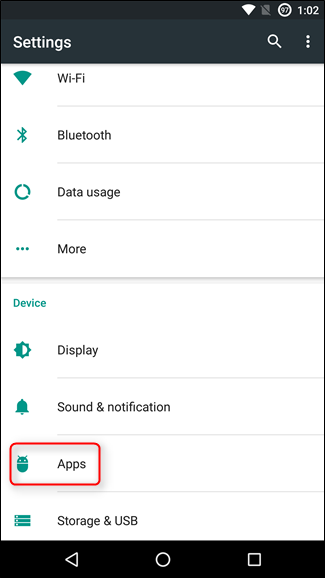The image is a screenshot captured in portrait mode, with a specific section outlined in red. The upper left-hand corner to the upper right displays a black stripe. In the upper right-hand corner, there's a '97' inside a circle followed by '102'. 

The next row has a light black background and contains the word "Settings" on the left, alongside a search icon and three vertical dots on the right. The remainder of the screen transitions to a white background, organized into two distinct sections divided by a thin gray line.

The first section under "Settings" features four rows:
1. Wi-Fi
2. Bluetooth
3. Data Usage
4. More

The next section is under the "Device" category, which is highlighted, with its label in teal font. This section also contains four rows:
1. Display
2. Sound & Notification
3. Apps
4. Storage & USB

The creator of the screenshot has specifically highlighted the "Apps" row by drawing a red border around it. The "Apps" row includes an icon that resembles a small bug. The highlighted section emphasizes the steps needed to navigate: starting from the "Settings" menu, proceed to the "Device" category, and then select "Apps" from the third row.